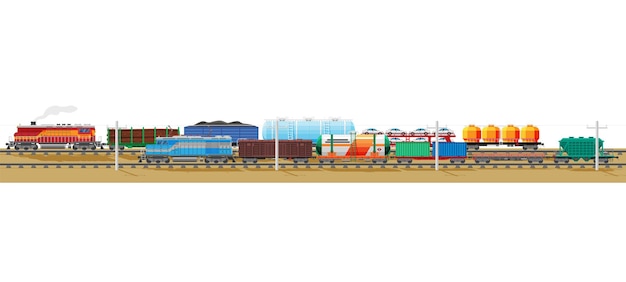This cartoon-like computer-generated image features a detailed scene of two freight trains traveling from right to left on parallel tracks, set against a clean white background with no borders. The ground beneath the tracks is a sandy beige color, and there's a series of white signal poles along the tracks.

In the foreground, the train has a blue and gray locomotive followed by a sequence of cars: a boxcar, a tanker car, and several flatbeds. The first flatbed carries two containers, one blue and one green, and the last flatbed holds a green container.

The second train, situated on the far track, has an orange and red diesel locomotive. It is hauling a varied load: a flatbed with planks, a boxcar filled with coal, a cylindrical tanker car, another flatbed with some vehicles, and a final flatbed carrying orange cylinders.

The overall effect is a wide, rectangular image emphasizing the vibrant colors and detailed arrangement of the train cars, which appear to float on the screen due to the unbounded white background.